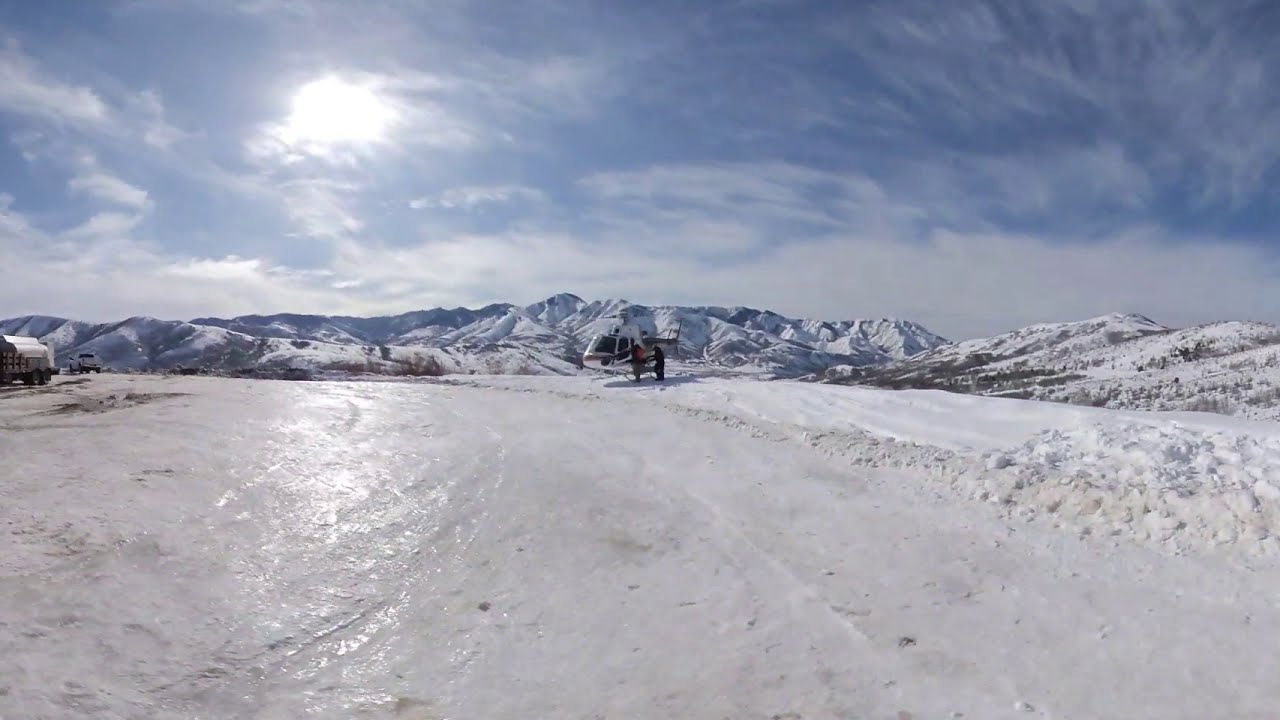Taken on a stunningly beautiful day, this image features a wintery outdoor scene with blue skies dotted by light, wispy clouds. The sun is subtly visible trying to poke through the clouds on the left-hand side. Dominating the background are majestic, snow-covered mountain ranges stretching across the horizon. The foreground showcases a smooth, icy road that curves from the right to the left, with densely packed snow glistening under the sunlight. 

A white helicopter is parked on a snowy patch towards the middle back of the image, with two people standing beside it, appearing to engage in conversation. Far off in the distance on the left, there is a white truck and a big-rigged vehicle or trailer accompanied by barrels. The entire composition encapsulates a serene yet dynamic winter landscape, emphasizing the vastness and beauty of the snow-covered surroundings.